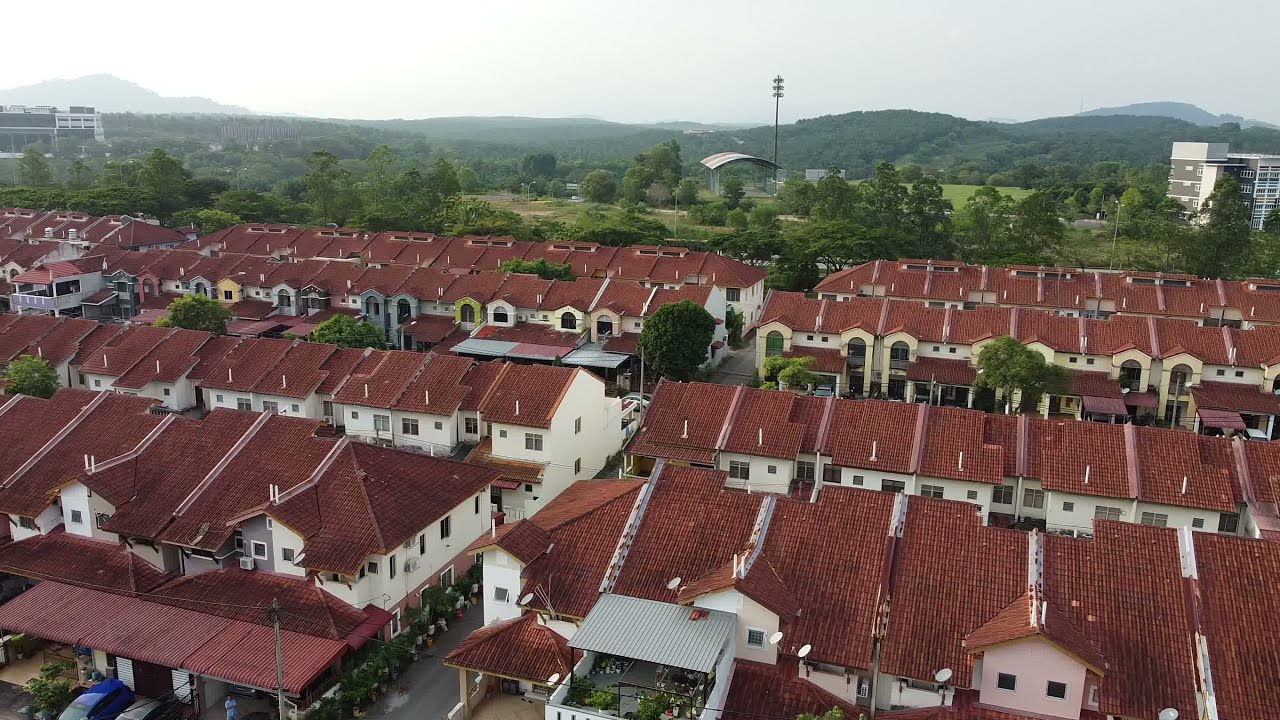The image is an aerial, photorealistic view of a tightly packed neighborhood, with the bottom two-thirds occupied by long, connected buildings featuring multicolored facades—primarily white, cream, and other shades—housing multiple properties. The roofs of these buildings are uniformly covered in terracotta or reddish adobe tiles, creating a striking orangey-amber hue. A diagonal gray asphalt road cuts through the neighborhood near the center, partially obscured by the buildings, and is marked by the presence of a blue car in the bottom left corner. Interspersed among the buildings and along the road are vibrant green trees, contributing to the lushness of the scene. 

In the distance behind the neighborhood, dense forests and a mixture of bright green foliage add a rich backdrop. Further back, a range of rolling hills and mountains, densely covered in greenery, stretch across the horizon, fading from vibrant green to a hazy tone as they recede. Prominent gray or white multi-story buildings flank both the right and left sides of the image. A distinctive large canopy, supported by arches and crowned with a tall pole featuring some sort of structure at the top, is noticeable further into the background. The sky is a light gray, brighter on the left side, indicating the presence of sunlight filtering through the hazy atmosphere.